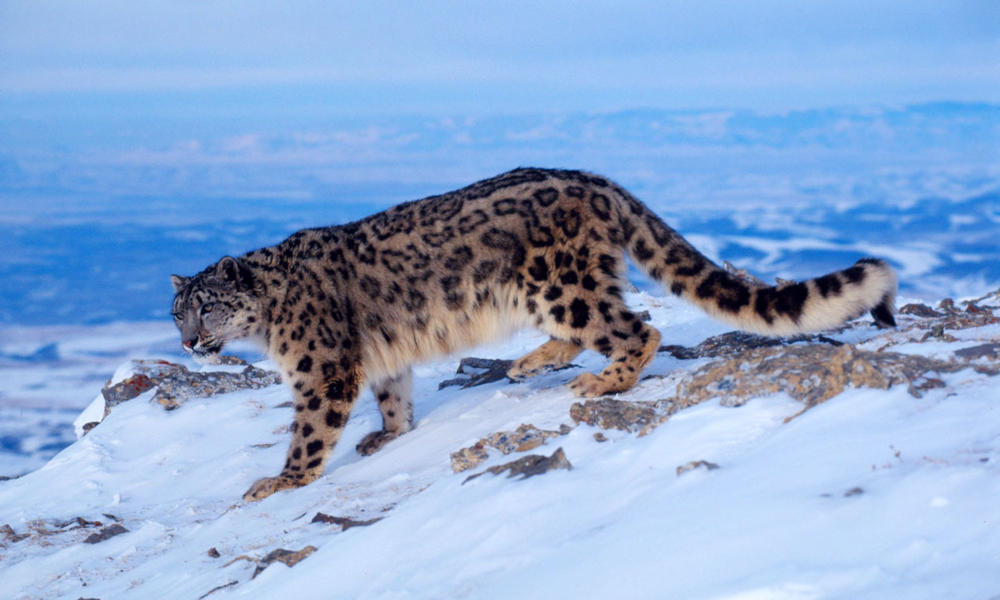In this vivid nature photograph, a snow leopard, distinguished by its large, muscular body and long, thick tail, is captured walking on a rocky, snowy surface high in the mountains. The snow leopard's yellow fur is patterned with distinctive black spots, giving it a leopard-like appearance. The photo presents a side view of the majestic animal, but its head is turned just enough for its two piercing eyes to gaze directly at the viewer, conveying a sense of intensity and presence.

The rugged terrain and stark winter conditions are evident, with the snow leopard appearing to traverse a descending slope. The scene's colors primarily feature the cool blues and whites of the snow and sky, contrasted by the tan and black hues of the leopard's fur. The background reveals a sweeping, snowy landscape far below, suggesting that the photograph was taken at a significant altitude, where the land drops away into a distant valley. The image, devoid of any textual elements, captures the raw beauty and harshness of nature, highlighting the snow leopard's adaptability and resilience in its frozen, mountainous habitat.